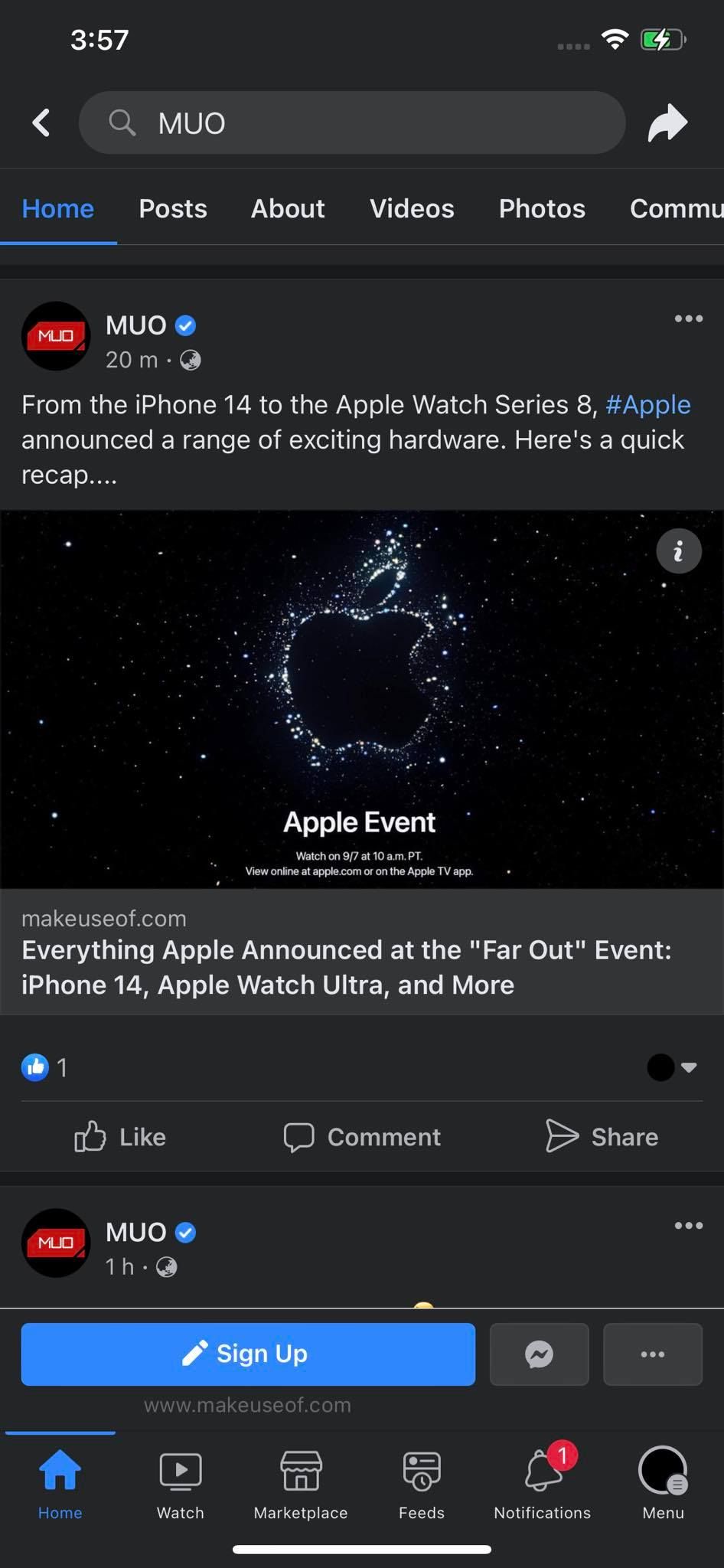The screenshot is taken on an iPhone, as indicated by various on-screen elements typical of iOS. The background is a dark gray shade. At the top of the screen, the time reads 3:57, flanked by a full Wi-Fi signal indicator to the right and a battery meter displaying approximately 60% charge. Centered on the screen is an ad for an Apple event, prominently featuring the Apple logo styled as a constellation made of stars, with a void forming the shape of the apple and its leaf, surrounded by clusters of stars that diminish as they radiate outward.

Beneath the advertisement, there is a search field with "MUO" typed into it. Below this, a navigation bar shows tabs labeled "Home," "Posts," "Videos," "Photos," and "Community," with "Home" highlighted in blue. The current feed includes a post from MUO, identified with a blue check mark. The post title reads: "From the iPhone 14 to the Apple Series 8: Apple Announces a Range of Exciting Hardware. Here's a Quick Recap." Additionally, the thumbnail for the post includes the Apple event's details: "Apple Event - Watch on 9/7 at 10 a.m. Pacific Time. View online at apple.com or on the Apple TV app."

A makeuseof.com announcement is also visible, titled "Everything Apple Announced at the Far Out Event: iPhone 14, Apple Watch Ultra, and More." This post has received a thumbs-up, with options to like, comment, and share. Below this is another post by MUO from one hour ago, while the post about the Apple event was made 20 minutes ago. At the bottom of the screen, there are six icons for navigating different sections: "Home," "Watch," "Marketplace," "Feeds," "Notification," and "Menu".

Overall, the screenshot captures an iPhone interface showcasing user interactions and notifications of a recent Apple event.